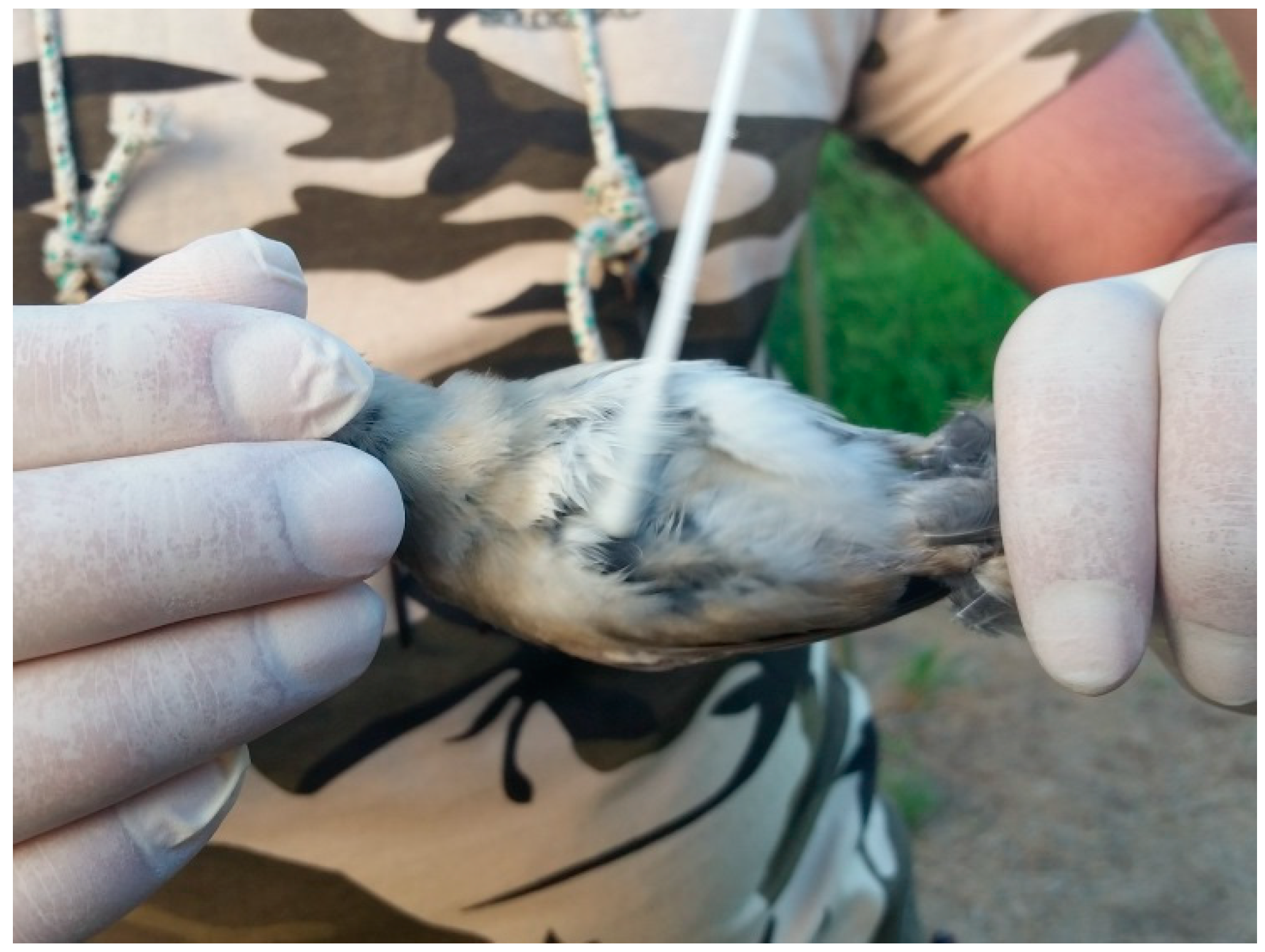The color photograph depicts a close-up of an individual, likely a conservationist or researcher, dressed in a green, beige, black, and brown camouflage-patterned shirt. They have a blue-and-white cord or rope around their neck and are wearing white rubber gloves. The person is gently holding a small bird with a bluish-brown, gray, and black plumage, and a white underbelly, carefully cradling it such that its head and wings are not visible, suggesting it might be on its back. The background features a blurred stone path with green grass. Another person's arm can also be seen near the main subject, adding to the impression of a fieldwork or research setting.